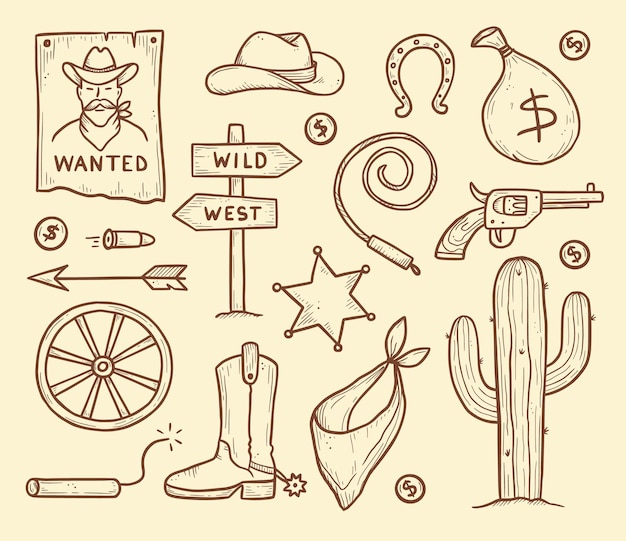The image features a cream-colored background adorned with a variety of cartoonish, dark brown drawings representing iconic symbols of the Wild West. Positioned in the top left, there's a wanted poster depicting a cowboy with a hat, a large mustache, and a bandana around his neck. To the right, you find a simple cowboy hat, followed by an upside-down horseshoe dotted with nail holes. Scattered around, there are multiple coins marked with a dollar sign, a coiled rope resembling a lasso or whip, and a Wild West directional sign with arrows pointing in opposite directions.

A bag of money tied at the top, a pointed arrow, and a six-shooter pistol with a wooden handle appear alongside a cactus with two arms. Additionally, there’s a classic sheriff's badge shaped like a six-pointed star. Towards the bottom left, a wagon wheel sits next to a stick of dynamite with a sparking fuse, a cowboy boot with a spur, and a tied bandana. There’s also a bullet illustrated to appear in motion, a simple bow and arrow, and a firecracker. The imagery is scattered across the entire poster, with all drawings retaining the beige background color within their dark brown outlines.